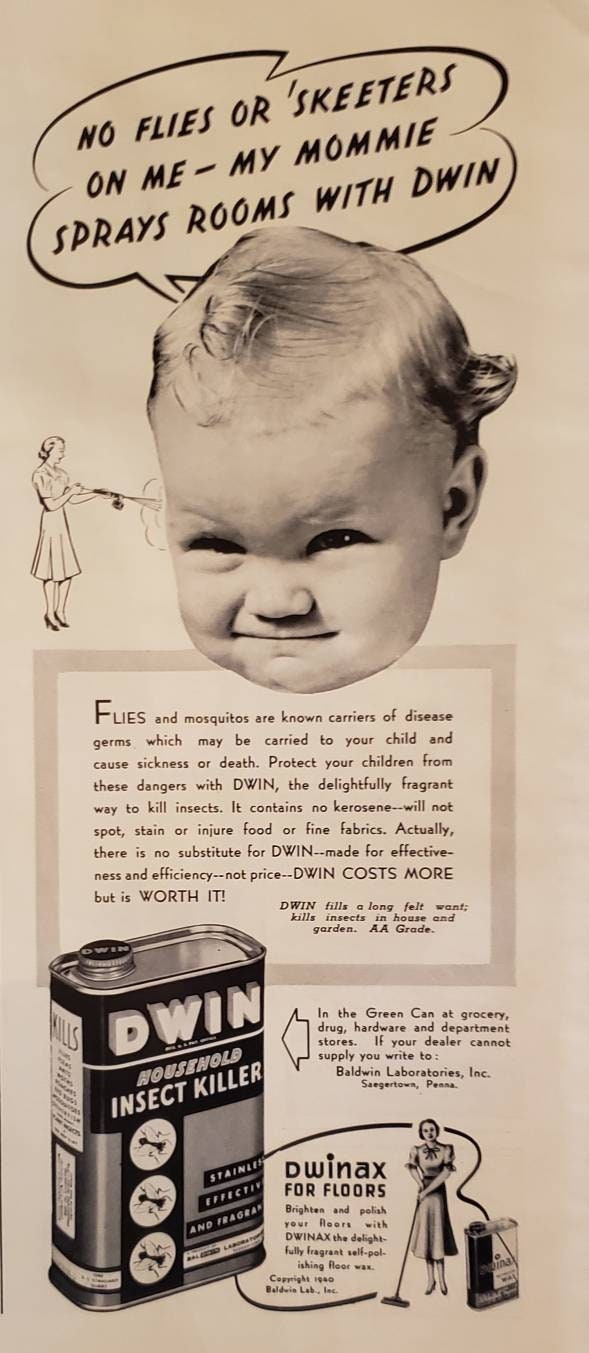This image is a black and white vintage advertisement, likely from the early to mid-20th century. It promotes DWIN, a household insect spray. Central to the ad is a photograph of a baby's head with an expressive face. Above the baby, a speech bubble reads, "No flies or skeeters on me. My mommy sprays rooms with DWIN." A woman in a dress is illustrated spraying the insecticide nearby. Beneath this central image, there's a detailed description emphasizing the dangers of flies and mosquitoes as carriers of disease germs, advocating DWIN as a safe and effective solution. The text highlights that DWIN is free from kerosene, will not spot, stain, or damage food or fabrics, and is superior in quality despite its higher price. The advertisement also features an image of a metal can of DWIN household insect killer, which can be found in grocery, drug, hardware, and department stores. If unavailable locally, consumers are directed to contact Baldwin Laboratories, Inc. Additional graphics include a woman using a mop and a promotion for DWIN wax for floors, which promises a fragrant, self-polishing finish. The ad concludes with the company’s information: Baldwin Labs, Inc.